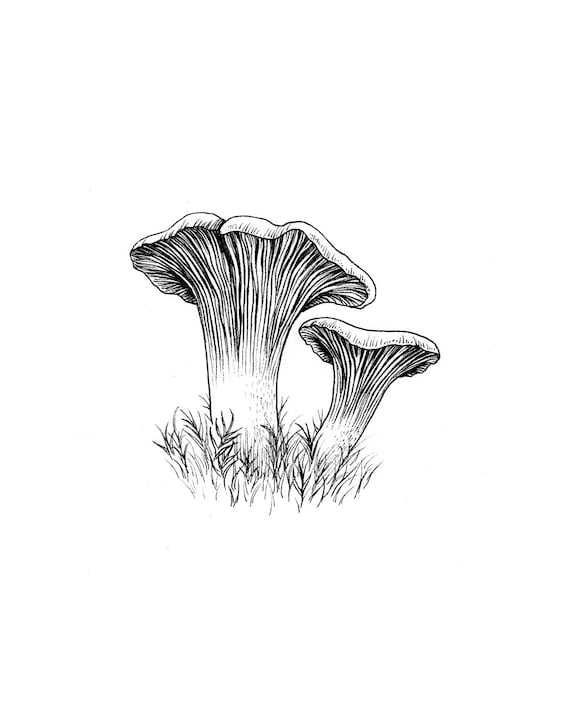The image is a simplistic yet detailed black and white computer sketch drawing with no border, set against a pure white background. At the bottom of the image, there is a small clump of wispy, straight blades of grass, each with offshoots. Emerging from this grass are two prominently featured mushrooms. The mushrooms have cylindrical stems that are completely white in their lower halves, with dark black lines extending from the heads downwards. The mushroom on the left is taller, wider, and has a straighter stem, while the one on the right is shorter and curves as it ascends. Each mushroom cap is characterized by its flat top with curvy, wavy edges that fold down towards the ground. The detailed sketch emphasizes the textural contrast between the grass and the mushrooms, with the latter's curving lines adding an intricate, dynamic element to the otherwise simplistic image.